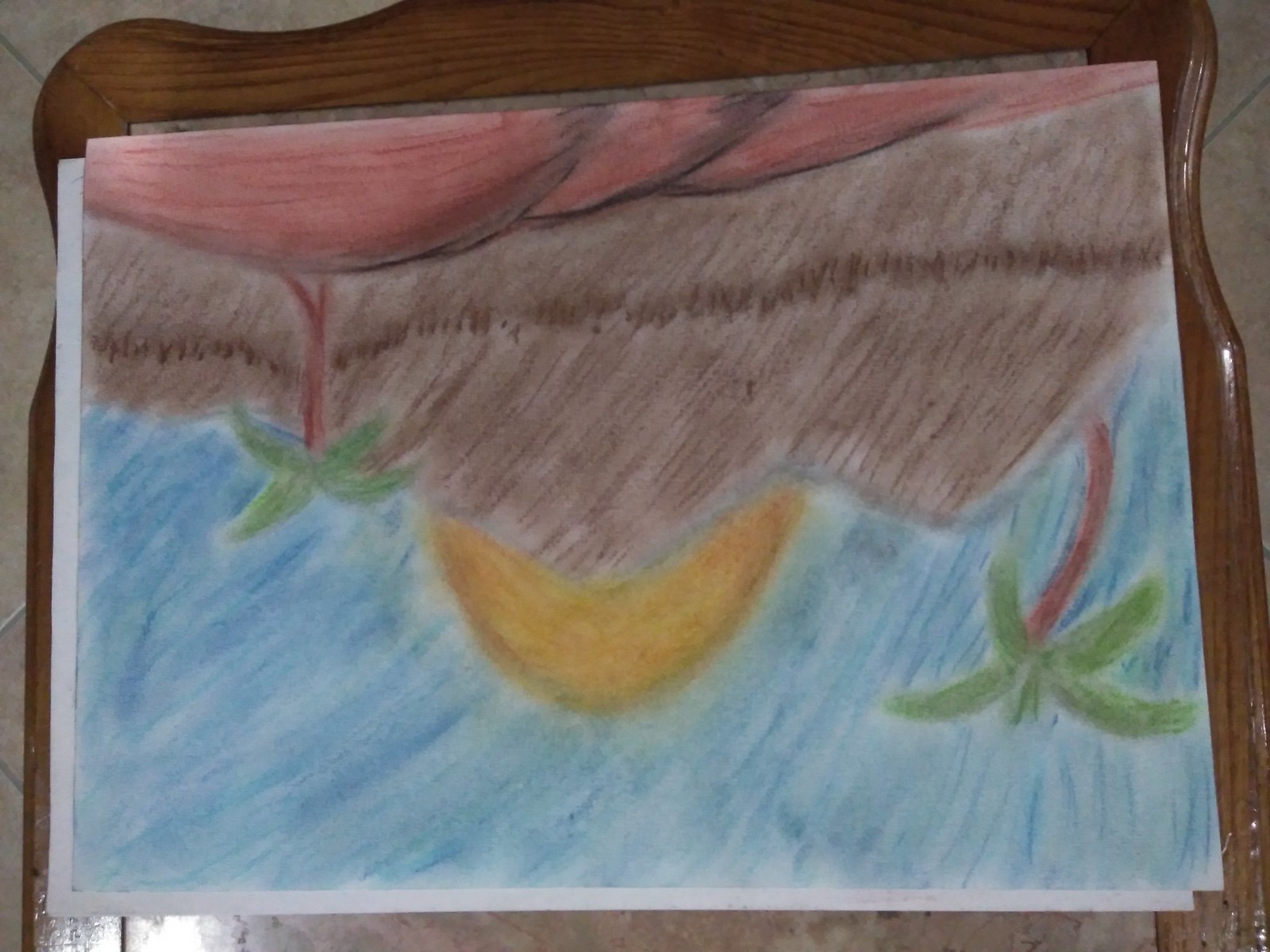This is an upside-down image of a child's drawing, possibly created with colored pencils or crayons, resting on a dark brown wooden surface. The primary focus is a large brown mountain or island with two palm trees on either side. The mountainous landscape features several red humps in the foreground, resembling a red beach or low-lying hills. Behind the mountain, a yellow semi-circle, representing the sun, protrudes into a sky that's fully colored in blue, likely done with a blue colored pencil. The palm trees have brown trunks and green fronds, with some trunks appearing slightly reddish and curved. Beyond the main drawing, another sheet of white paper is partially visible, hinting at an additional drawing underneath. The wooden surface supports the drawing, and the edges of the image reveal bits of a tiled floor, along with what appears to be a traditional wooden mirror frame in the background.